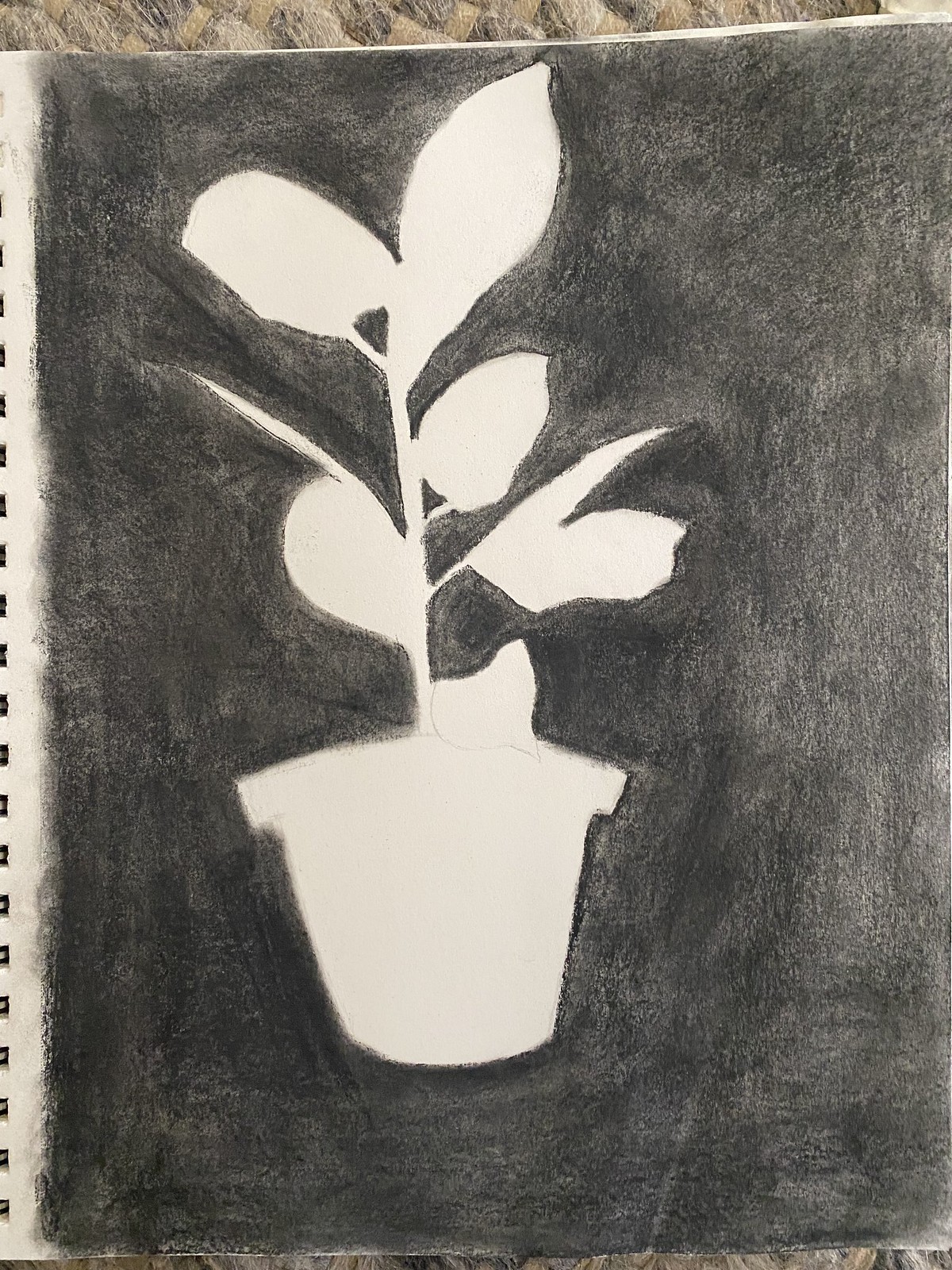This illustration features a plant pot depicted using negative space, giving it a unique and abstract appearance. The pot itself is not drawn but is instead implied by the absence of marks within a dark, densely shaded background. Rising from the center of this implied pot is a delicate stem, from which five leaves branch out. The surrounding area is filled in with a rich, black medium, possibly pencil or charcoal, which contrasts vividly with the untouched, pristine space defining the pot. This creative use of negative space emphasizes the minimalist yet striking form of the plant and pot.